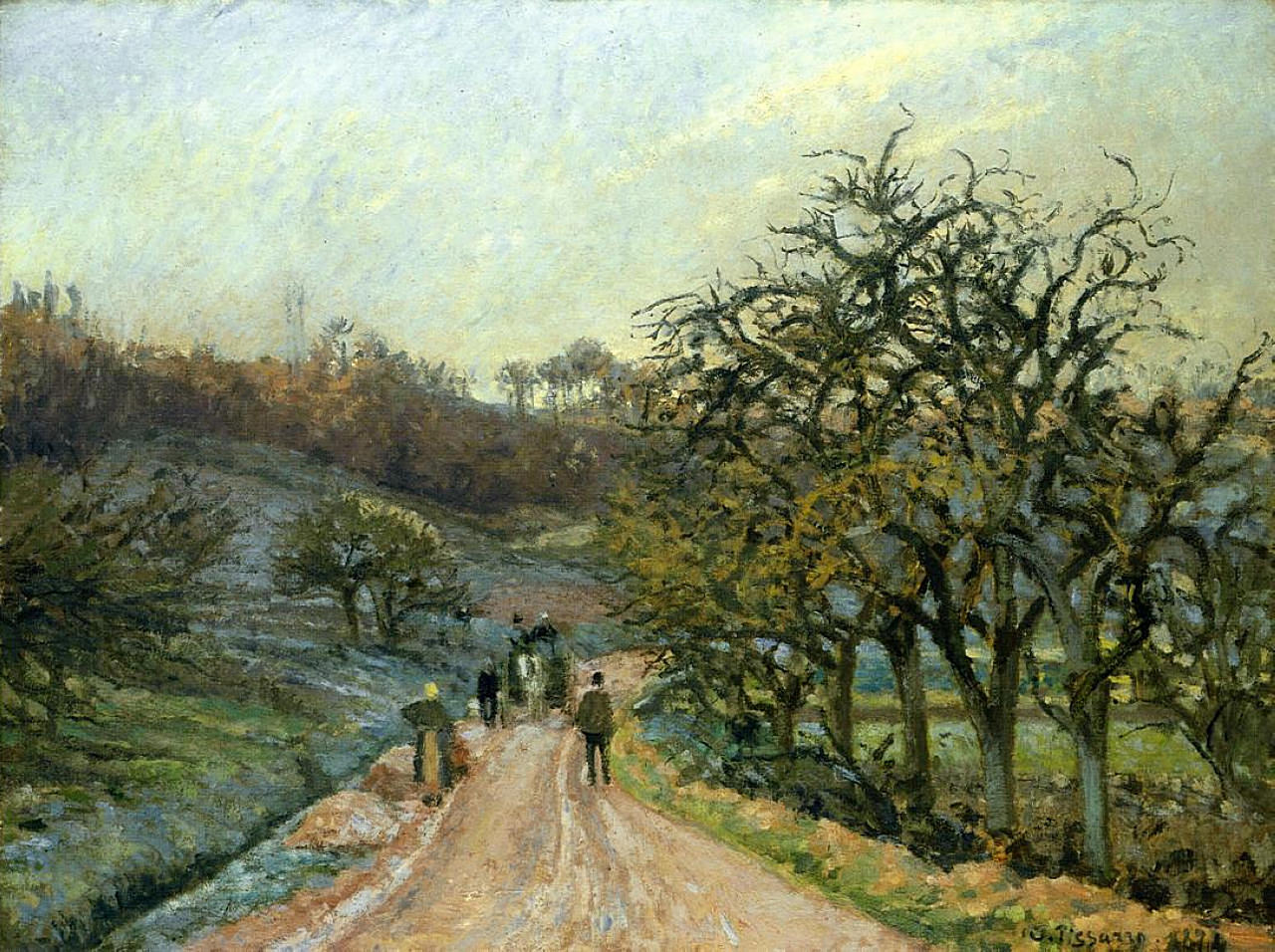This impressionist painting vividly captures a serene outdoor scene with meticulous detail. Dominating the composition, a beige dirt road meanders through the landscape, lined with trees bearing dark trunks and sparse, curly branches with mustard-green hues. On the right side of the path, these trees create a natural corridor, drawing the eye deeper into the scene. To the left, a hillside dotted with trees and bushes adds dimension with its palette of light blue, dark olive, lime green, and brown tones.

The sky above is predominantly blue with hints of misty clouds, painted in shades of white, yellow, and beige, indicating a bright yet slightly overcast day. Along the road, several human figures are depicted. In the foreground, a person dressed in all black walks alone, while a white horse-drawn carriage adds a touch of movement and nostalgia. Further back, two figures walk away from the viewer: one on the left in a yellow head covering and a green and tan robe, and the other on the right in a dark green jacket and black pants.

The overall color scheme harmonizes with the detailed landscape, where strong brushstrokes convey the texture and depth characteristic of the impressionist style. Notably, the artist's signature can be found in the bottom right corner, leaving a personal mark on this tranquil scene.